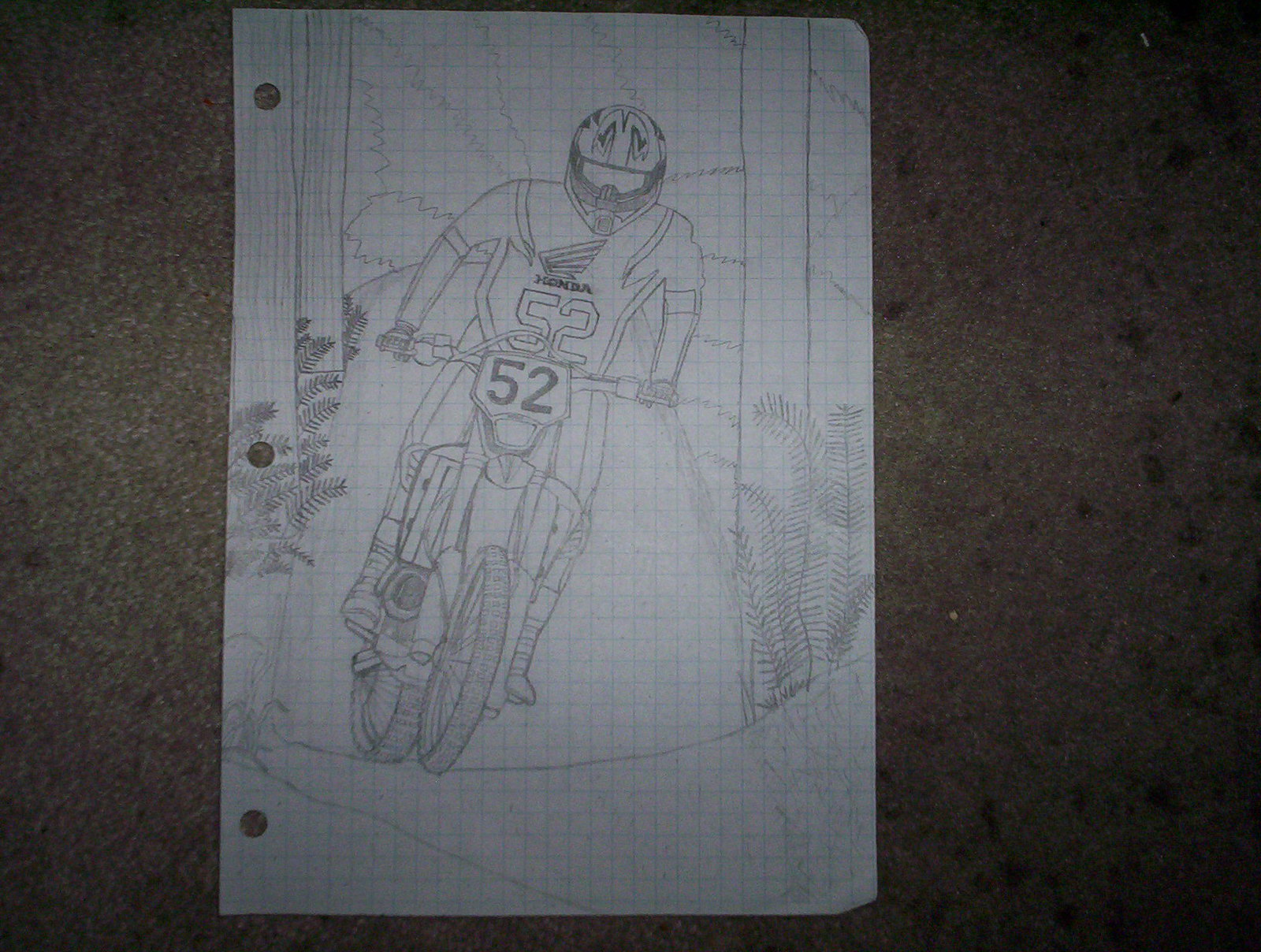The image is an illustration on graph paper, distinguished by the checkered blue lines and three punch holes along the left margin. The paper rests on a tan-colored, slightly dirty carpet with black and brown speckles. The pencil drawing depicts a man on a motorbike, wearing a long-sleeve jersey emblazoned with "Honda 52" and a helmet adorned with a fire pattern. The bike also bears the number 52. The rider's precise face is obscured by the helmet's visor. He is navigating through a wooded area, with visible tree trunks, pine trees in the background, and fern-like plants on either side. The rider appears to be tilting slightly to his left (right for the viewer) as he traverses a hilly path.